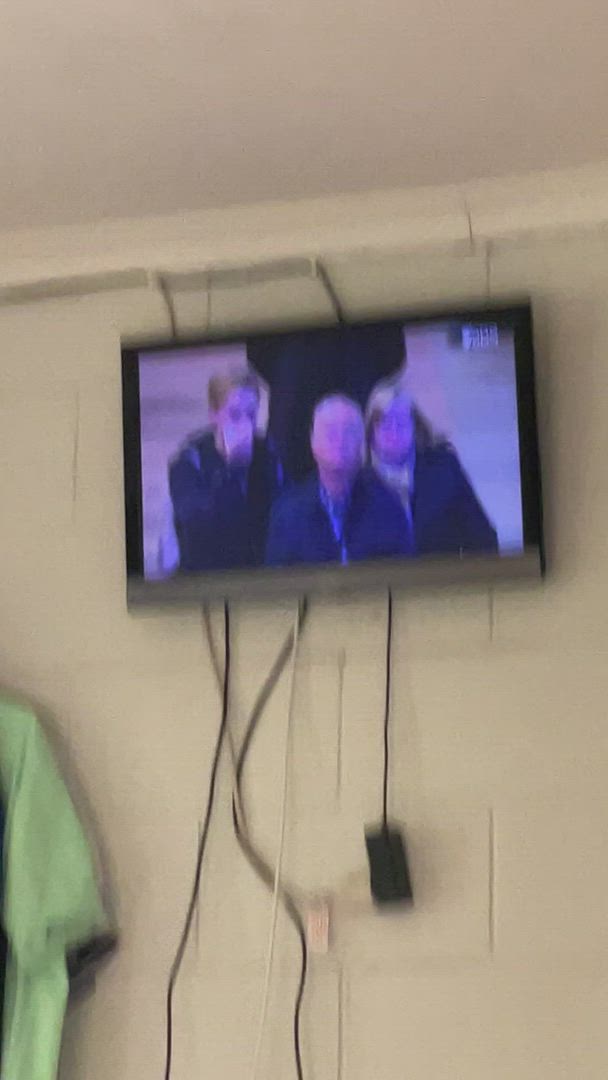The photograph depicts a small flat-screen television, likely around 32 inches, mounted high on a white cinder block wall. The picture quality is somewhat blurry, obscuring the finer details of the program. On the television screen, there are three visible figures: a man in a blue jacket and shirt stands in the center, flanked by a younger man with reddish blonde hair and a blue jacket on his left, who seems to be holding his hand to his face, possibly speaking into a device or covering his mouth. To the right of the central figure stands an older woman with long gray hair, also dressed in a blue jacket. Their features are not entirely clear due to the blur. Below the television, a collection of wires hangs down, with a power plug connected to a socket just beneath the TV, though it seems somewhat disorganized. On the left side of the frame, the corner of a lime green short-sleeved t-shirt is visible, hanging from the wall. The setting suggests a utilitarian space, possibly a basement or warehouse-like environment, characterized by its plain white cinder block walls and simple decor.